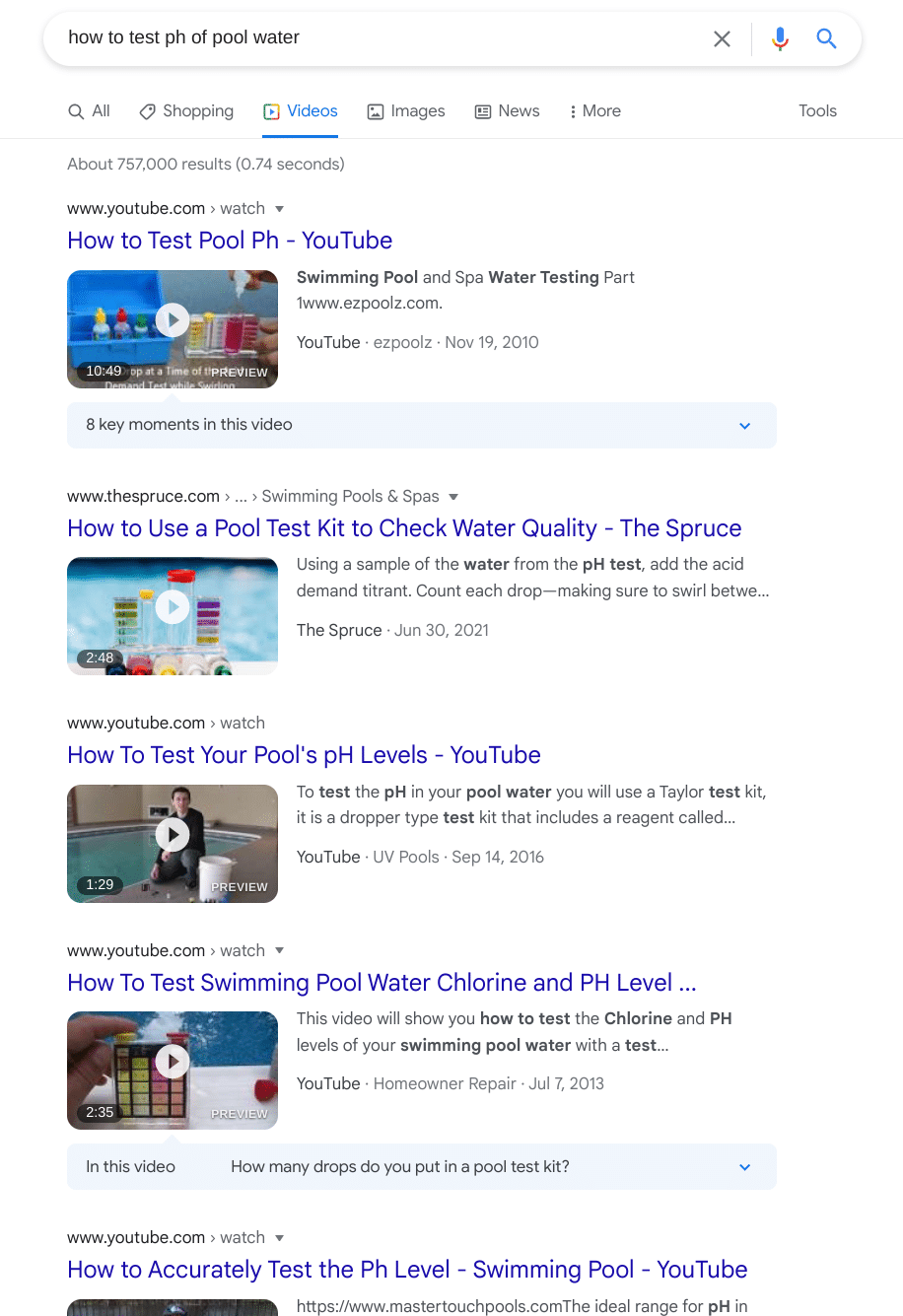In the image, a Google search page is displayed at the top, where the search bar reads "how to test pH of pool water." The iconic Google microphone, colored in blue, red, and yellow, and a magnifying glass icon for the search function are clearly visible. The 'All' tab, along with 'Shopping,' 'Videos,' 'Images,' 'News,' 'More,' and 'Tools' options, are present, with the 'Videos' tab being highlighted in blue and underlined. Beneath, it shows there are about 757,000 results found in 0.74 seconds.

The first search result is a YouTube video titled "How to Test Pool pH." The preview includes a screenshot featuring a colorful blue box with yellow, red, and blue bottles used for testing, alongside a clear container with water to measure the color change. This video, originating from "www.epools.com," is titled "Swimming Pool and Spa Water Testing Part One" and was posted on November 19, 2010. Below this, there are additional video search results with corresponding screenshots displayed.